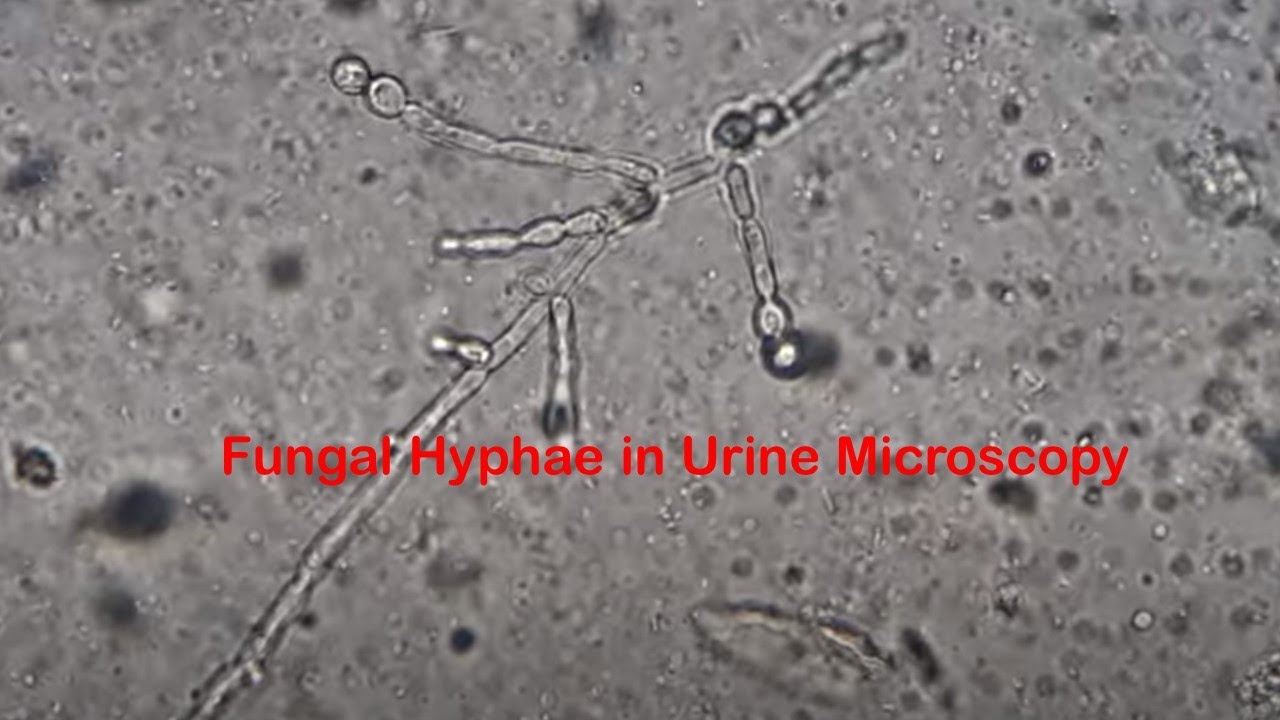This grayscale microscopic close-up image shows fungal hyphae in a urine sample, as indicated by the red text "fungal hyphae in urine microscopy" across the middle. The central structure, resembling a branched plant stem, extends from the lower left to the top center of the image. This straw-like formation features six distinct branches: three extending to the left, two to the right, and one continuing upwards. Scattered throughout the background are variously sized splotches and dots, giving the image a textured appearance reminiscent of a lunar surface. The overall context and labeling confirm the presence of fungal elements in the urine sample.